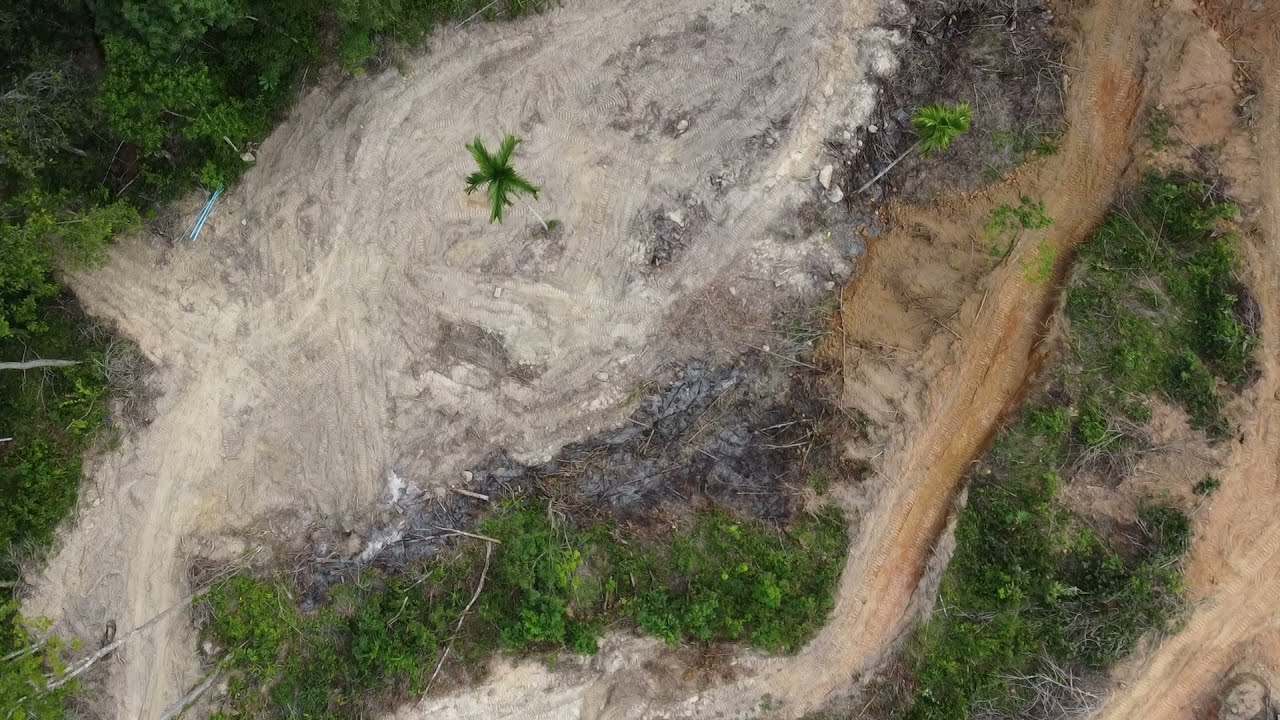This is an aerial, top-down view of a clearing in a naturally forested area, likely impacted by a natural event such as a fire or flood. The upper left diagonal half of the image features a light-colored sandy clearing with a lone green palm tree at its center, surrounded by a backdrop of greenery at the outermost corner. The right third of the image contrasts with brown compacted soil, potentially clay, and is framed by further shrubbery. Notably, a rural-looking, dirt path weaves through this section, adding to the sense of a landscape recently scarred by a natural calamity. The image is devoid of any human presence, vehicles, or structures, emphasizing the solitary and untouched nature of the scene. Speculated traces of ash on the ground further hint at a fire having swept through, leaving behind this stark and quiet landscape.